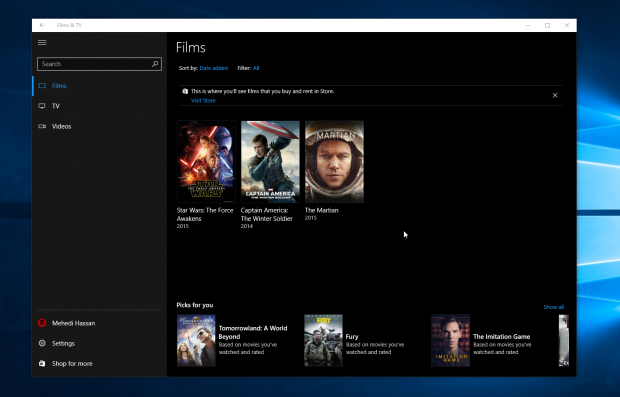This image depicts a detailed screenshot of a desktop application, possibly a media player or digital library interface, showcasing its layout and content organization. The screenshot is primarily occupied by a window with a white bar at the top, which includes a back arrow on the left and minimize, maximize, and close buttons on the right. The top of the window features the title "Films & TV" in gray text.

On the left side of the window, there is a vertical gray sidebar containing a menu button and a search bar at the top. Below the search bar, the text "Films" is highlighted in blue, indicating it as the selected category, with corresponding blue highlight bar next to it. Other categories, namely "TV" and "Videos," are listed below but not currently selected. Further down, the sidebar lists additional options such as a user name, "Settings," and "Shop for more."

The main content area on the right side has a darker background and displays the word "Films" in white text at the top. The lower section of this area is segmented into several parts. The upper portion displays three movie thumbnails: "Star Wars: The Force Awakens," "Captain America: The Winter Soldier," and "The Martian."

Further down, there is a section labeled "Picks for You," each entry accompanied by a thumbnail image and some descriptive text. The recognizable entries include "Tomorrowland: A World Beyond," "Fury," and "The Imitation Game." The text continues beyond the visible screen area, with a blue link possibly offering an option to "See More."